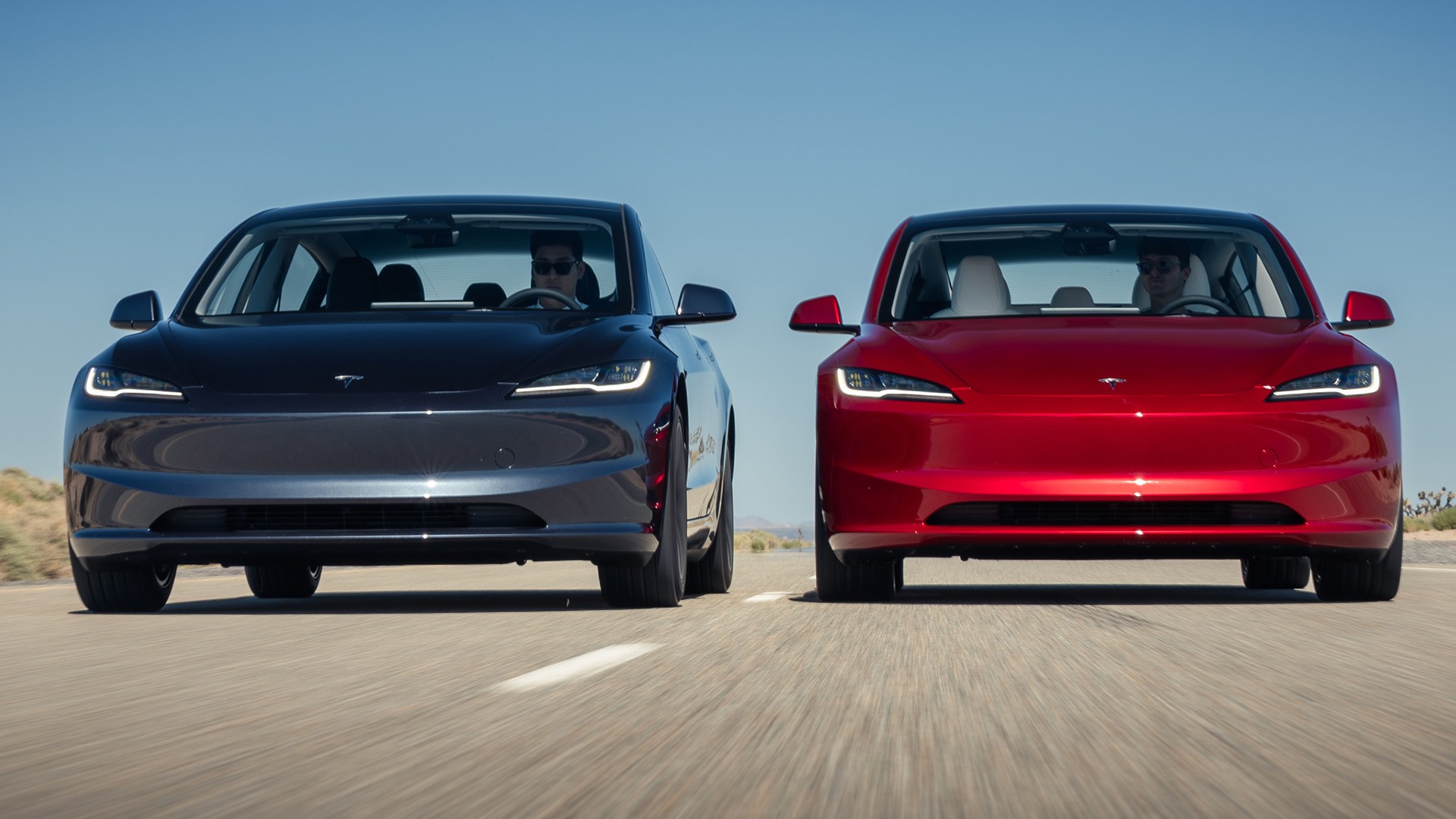In a vibrant and meticulously detailed photograph, two shiny Tesla sedans—a red one on the right and a blue one on the left—drive side-by-side down a gray, asphalt two-lane road marked by a white dotted center line. Captured from a low, almost road-level angle, the image emphasizes the glossy, reflective finish of the vehicles, suggesting digital enhancement for an ad-like perfection. Both cars, likely Model S, show distinct interior details: the red Tesla boasts a white interior, while the blue one has a darker one. The drivers, who appear to be male and wear sunglasses, are mostly indistinct but add a human element to the scene. The landscape in the background reveals a desert-like environment with hints of green and beige grasslands under a flawlessly blue sky, void of clouds, emphasizing the pristine and streamlined aesthetic of the photograph.